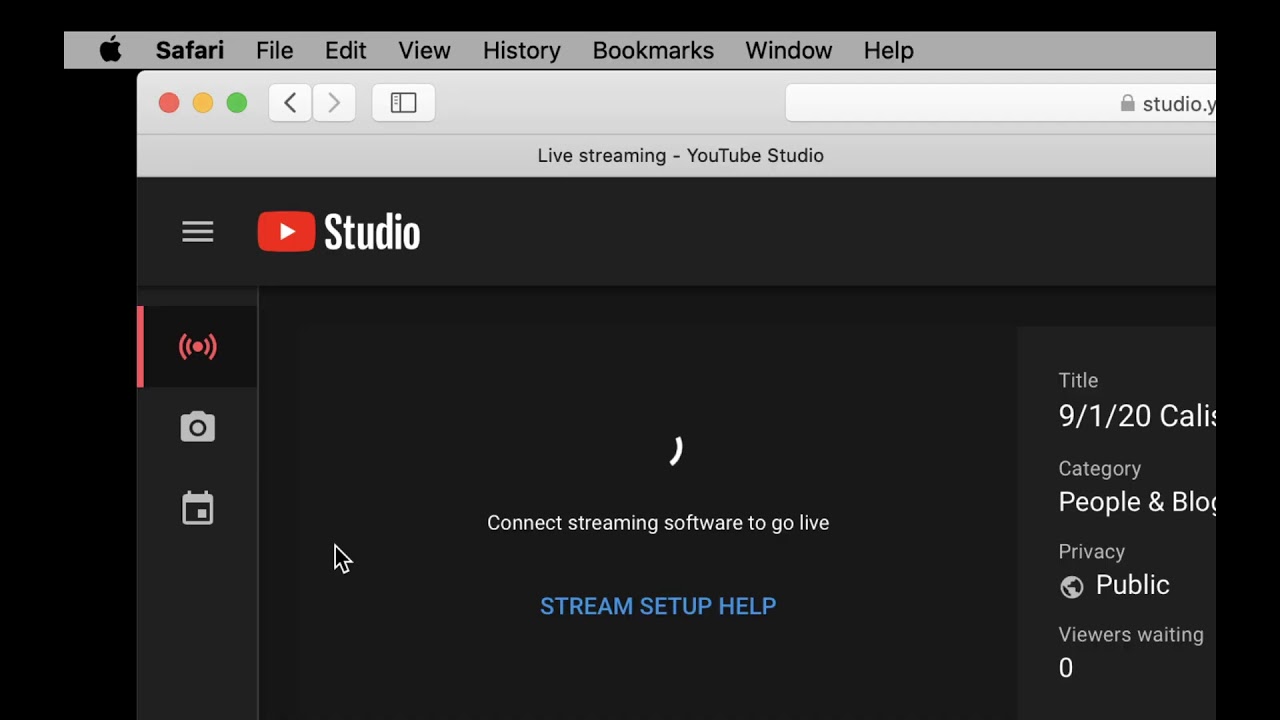The image consists of a black rectangle with a gray banner at the top. Centered within the gray banner is an Apple logo, followed by menu options: Safari, File, Edit, View, History, Bookmarks, Window, and Help.

Below this, there is a lighter gray rectangle containing three circles (red, yellow, and green) on the left, typically representing window control buttons. Adjacent to these circles are a left-pointing white arrow and a right-pointing white arrow, each inside a white square. There's also a white rectangle containing a black-bordered rectangle with a vertical line and dots at the left-hand side.

Further down, the text "Studio" is partially visible on a blocky interface element. Below this, it reads "Live Streaming - YouTube Studio." Another gray rectangle contains three parallel lines stacked vertically, and there's a red rectangular button featuring a right-pointing arrow and the word "Wait."

To the left, a red line runs down the image, leading your eye to a black rectangle with a dot flanked by two semicircles—likely indicating a playback button. Below this is a gray camera icon, followed by a gray calendar symbol.

In the center of the image, a white curved line appears alongside the instruction, "Connect streaming software to go live." Beneath this, "Stream Setup Help" is displayed in blue text.

On the right-hand side, the text "Title 9/1/20" is partially visible, alongside a cut-off word. The category "People and Blogs" appears, with "Blogs" partially obscured. The privacy settings show a globe icon labeled "Public," and indicate that there are zero viewers waiting.